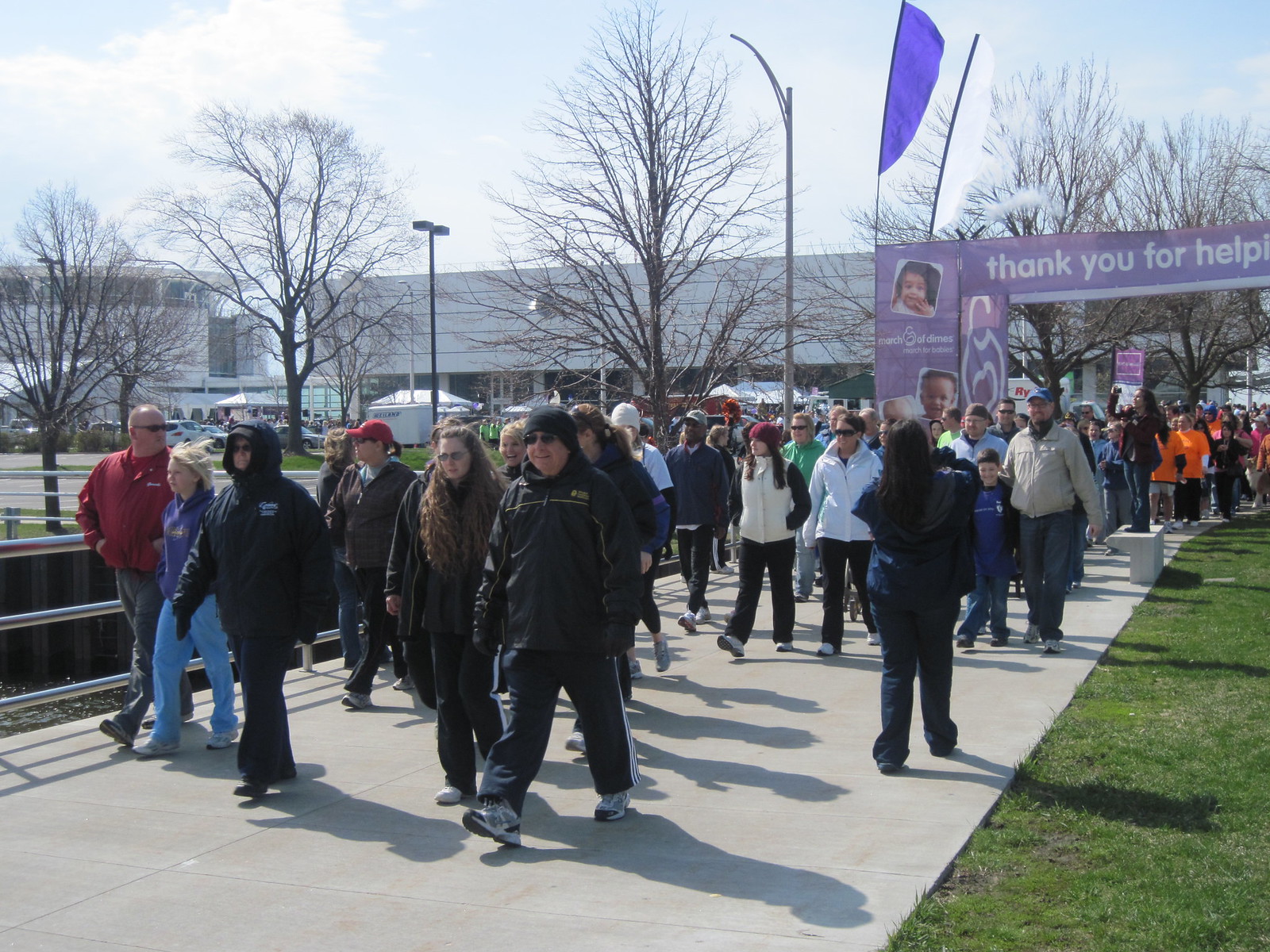This image depicts a bustling charity march taking place outdoors in the middle of the day. A large group of over a hundred individuals, dressed in heavy winter clothing, traverses a wide stone sidewalk. To the right of the sidewalk, a strip of green grass is visible, while on the left, a railing lines the path. In the upper right corner, there's a prominent archway bearing the message, "Thank you for helping," written in white on a purple background. Adjacent to this banner is a photo of a young girl on a pillar. The background reveals leafless trees, indicating a fall or winter setting, as well as several buildings, possibly a mall, streetlights, and a few tents. A diverse mix of people, encompassing various genders and races, walk in the center of the image. A single person is seen taking photographs of the event. The overall color palette includes greens, tans, blacks, light and dark blues, purples, reds, maroons, oranges, yellows, whites, and grays, reflecting the lively and varied atmosphere of this charitable gathering.